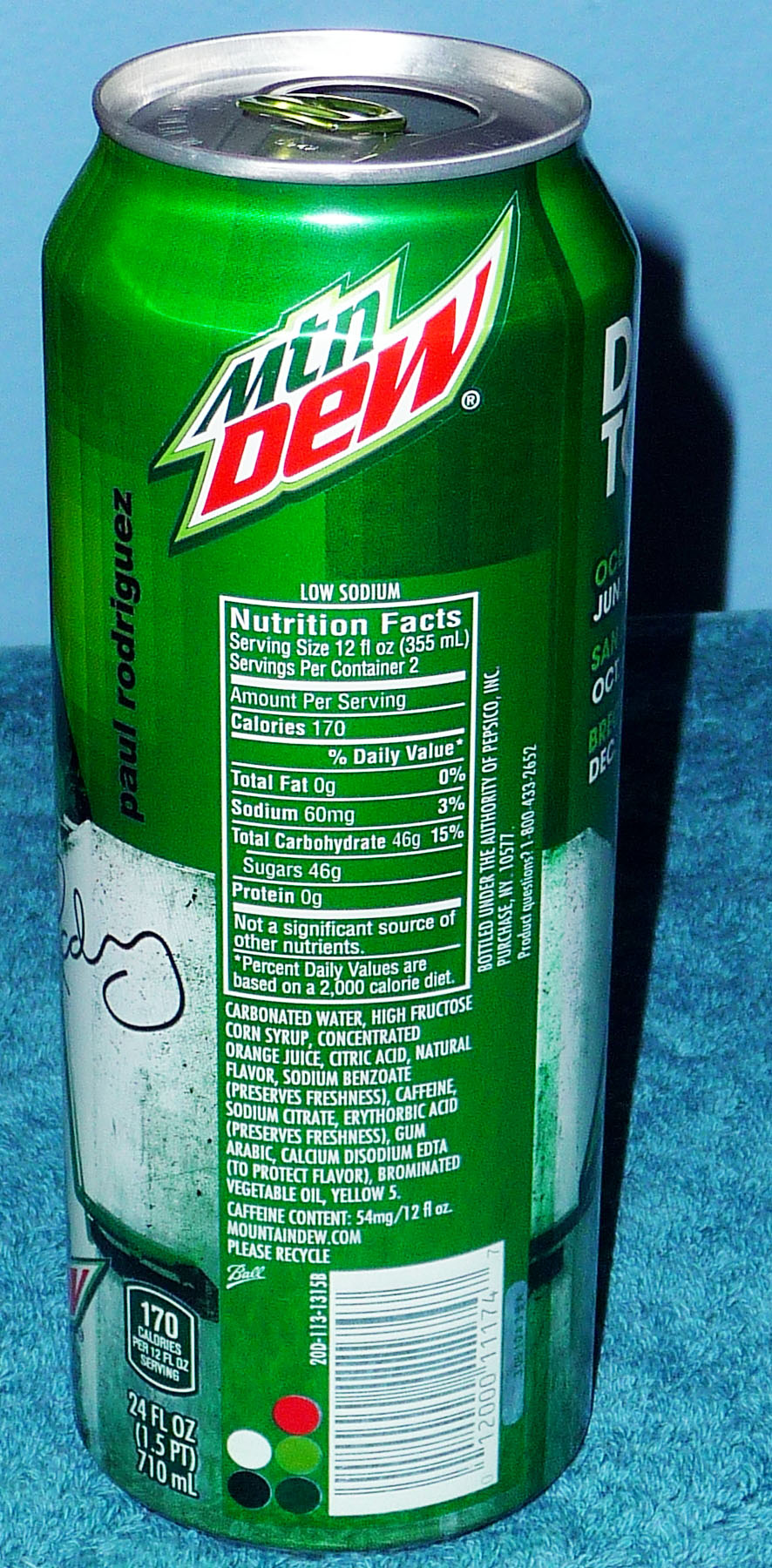This vertical, portrait-style photograph prominently features a large, close-up image of an aluminum can of Mountain Dew. The can occupies approximately 80-90% of the frame, drawing immediate attention with its vibrant green color set against the backdrop of a blue carpet and blue wall. The iconic Mountain Dew logo is clearly visible at the top of the can, while the lower portion displays the nutritional facts and ingredients, all printed in crisp white letters. Additionally, the barcode is also noticeable near the bottom of the can, completing the detailed visual composition.